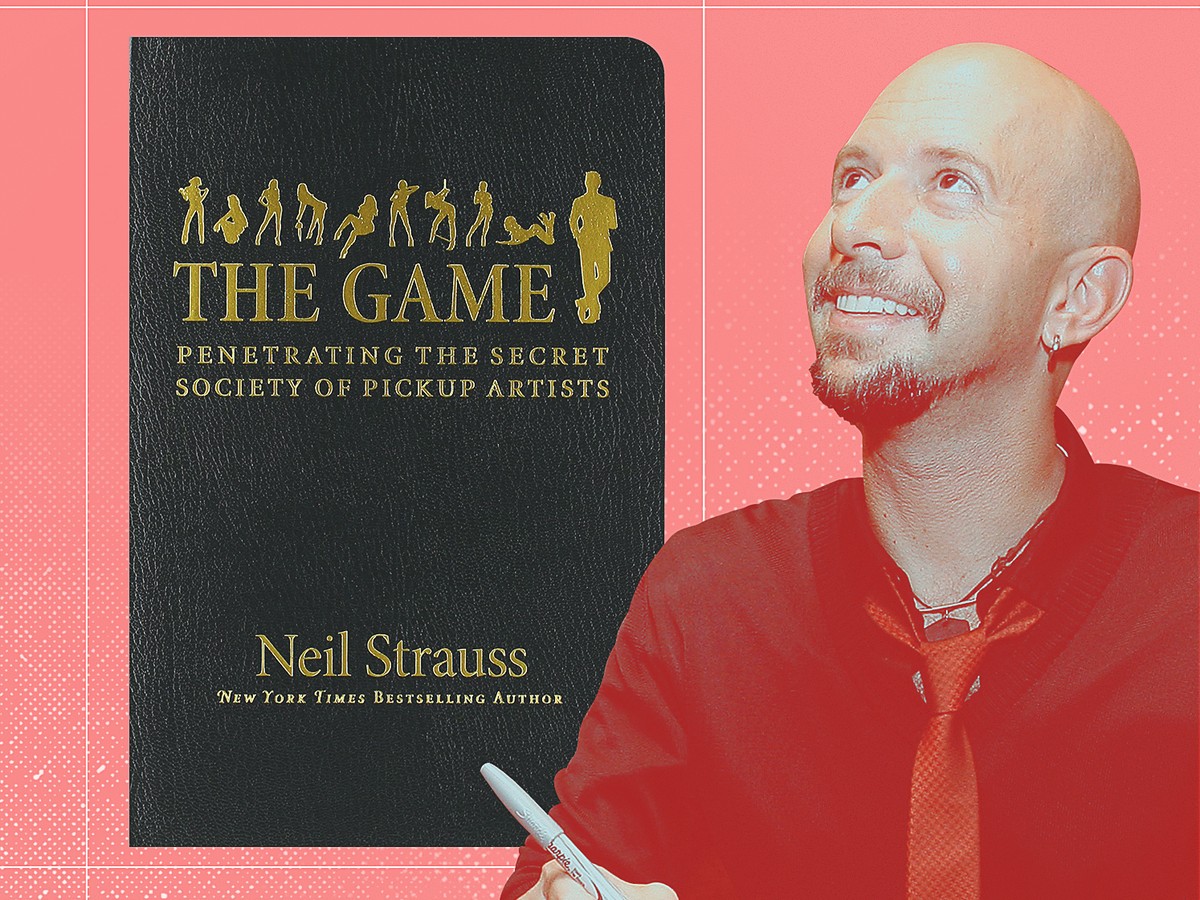The image depicts a bald man with a graying dark goatee and a mustache, wearing a loosely tied red tie over a black shirt that appears to have a red tint due to a filter applied over the image. He accessorizes with a silver necklace and a silver earring on his left ear. The man, who is looking up and smiling, is holding a Sharpie in his hand, suggesting he might be signing autographs. To his left, along the back wall, is a black leather-covered book titled "The Game: Penetrating the Secret Society of Pickup Artists" by Neil Strauss, a New York Times bestselling author. The book's title is written in gold print against the textured black leather cover. The background of the photo has a pinkish-red hue.